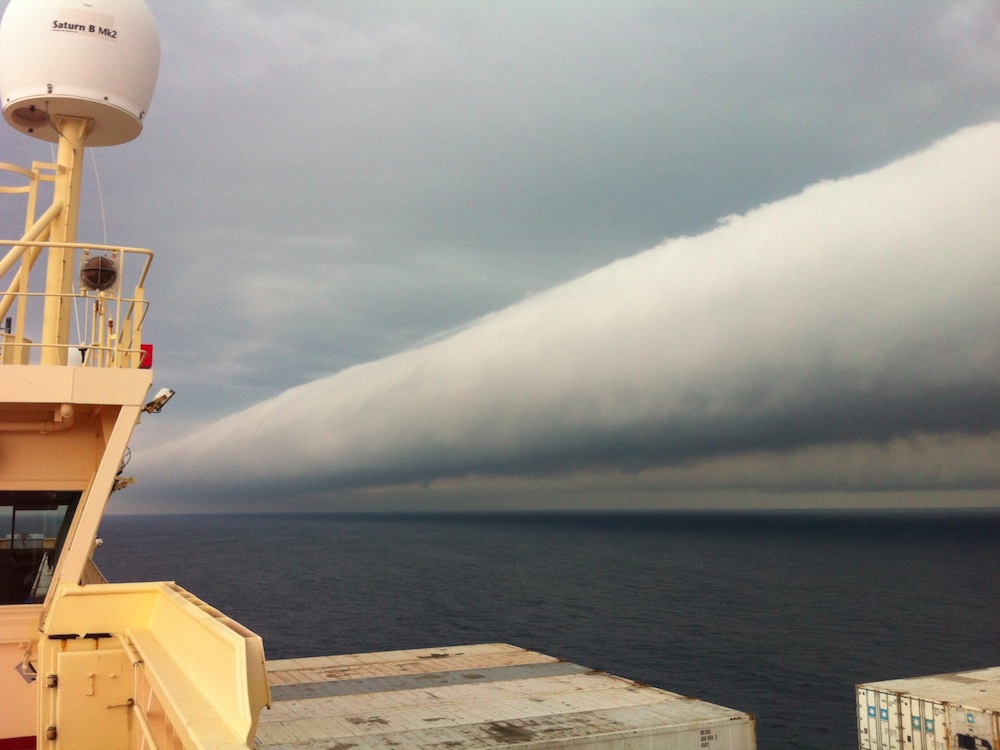The photo captures the side view from atop a freight ship, showcasing a complex metal structure on the left third of the image. This structure includes navigational equipment topped with a large white dome labeled "Saturn BMK 2", likely radar equipment. Beneath the dome is a yellow pillar, which is part of a scaffolding system and sidebars that extend downward. The structure also includes a railing, hinting at a nearby pilot's or captain's cabin, possibly the viewpoint of the shot. 

In the bottom right, the tops of shipping containers are visible. Beyond the ship's deck, the vast ocean stretches out into the distance. The water is a dark blue-gray, reflecting the ominous weather. Dominating the background is a dramatic storm front, characterized by a distinct line of cylindrical clouds. These clouds are white on top and dark at the bottom, casting a shadow over the ocean and creating a stark contrast between the clear sky to the left and the looming storm to the right. The overall scene conveys a palpable tension as the ship appears to be on the verge of sailing into the storm.